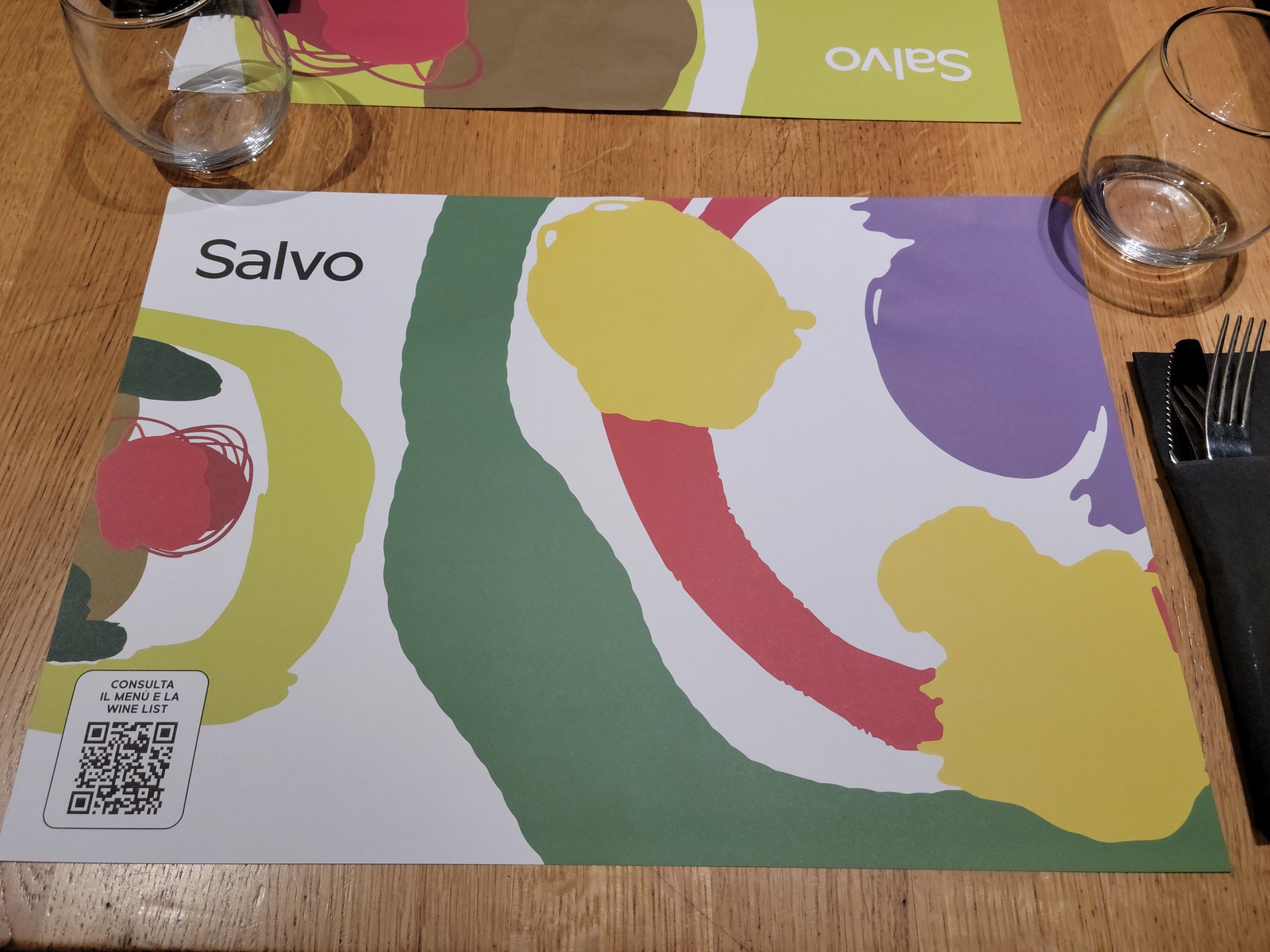This full-color photograph captures a detailed scene from a restaurant setting. Centered on a light brown wooden table is a vibrant, abstract placemat with a multitude of colors including browns, blacks, reds, greens, blues, yellows, purples, white, and pink. The design appears hand-painted and does not represent any particular object. In the top left corner of the placemat, the name "Salvo" is prominently displayed. Two clear drinking glasses are positioned at the upper corners of the image, while a knife and fork wrapped in a black cloth napkin rest on the far right side. Additionally, a QR code is visible in the bottom left corner of the placemat, inviting diners to consult the menu and wine list. The overall composition places these various elements in the center of the image, conveying a cozy and inviting indoor restaurant atmosphere.